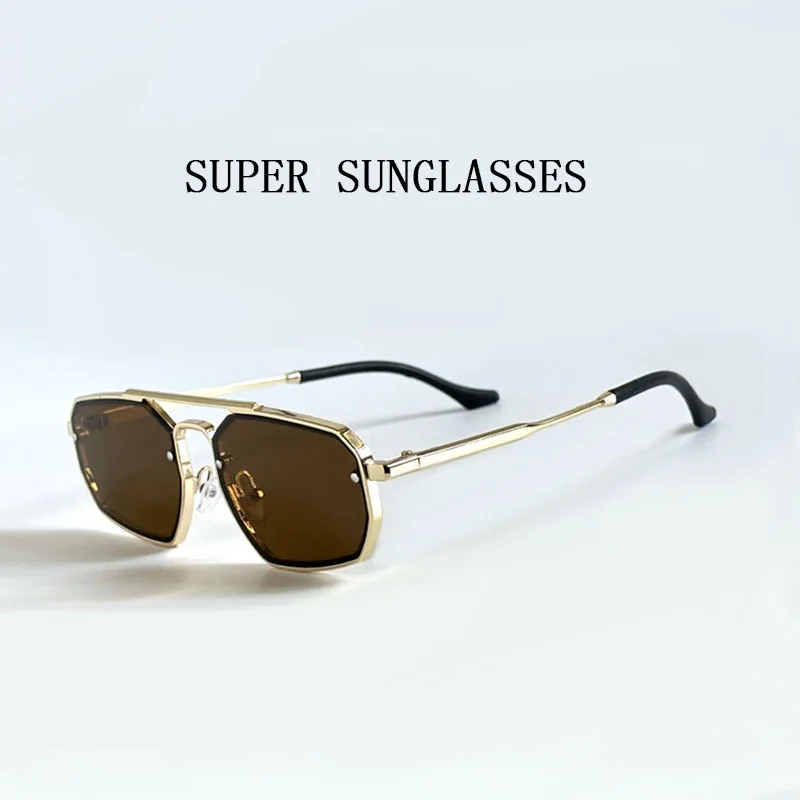The image showcases a sleek, modern advertisement for Super Sunglasses, designed in a squared aviator style. The background features a gradient from pale blue at the top, fading to white at the bottom, creating a subtle and visually appealing contrast. At the top center, "SUPER SUNGLASSES" is prominently displayed in bold, black, all-caps text. Below the text, the sunglasses are elegantly displayed, revealing their geometric, angular design with gold frames and black-tipped arms. The lenses exhibit a dark, translucent gradient from black to a brownish sepia tone. The image, square in format, likely mimics an Instagram post and exudes a luxurious vibe, further reinforced by the reflective, gold detailing and sharp, angular lines of the sunglasses. The sunglasses are resting on a white surface, casting subtle shadows that enhance the photograph's depth and realism.